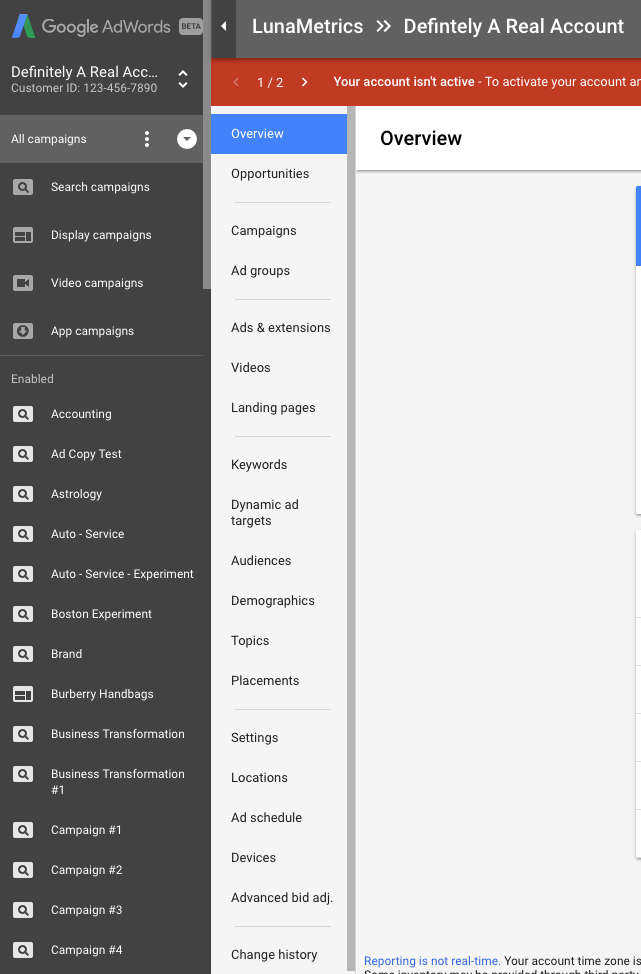A detailed screenshot from a web page showcasing the Google AdWords interface:

The left-hand side of the screenshot features a dark gray sidebar. At the top of this sidebar, there is a logo split into baby blue and green colors resembling an uppercase "A" without the crossbar. Below the logo, the text "Google AdWords" is displayed in gray.

On the upper right, there's a rounded rectangle shaded in mid-gray, containing the black capitalized text "BETA". Below this, in white text, it reads "definitely a real ACC" followed by an ellipsis. Directly beneath this, an up-and-down white arrow icon is present. Further down, the text "Customer ID" appears in gray, followed by a sequence "••• 123-456-7890".

Below the Customer ID, there’s a lighter gray section with white text displaying "All Campaigns", accompanied by three bold white ellipses and a bold white circle housing a downward-pointing gray arrow. A mid-gray square with a black magnifying glass icon is next, labeled "Search Campaigns" in mid-gray text.

Subsequent options include an icon resembling a newspaper, titled "Display Campaigns"; a video camera icon labeled "Video Campaigns"; and a microphone icon under a circle, named "Ad Campaigns". Below these, the text "Enabled" appears in gray, followed by multiple light gray squares containing black magnifying glasses. The list under these squares includes options in light gray text: "Accounting", "Ad Copy Text", "Astrology", "Auto-Service", "Auto-Service - Experiment", "Boston Experiment", "Brand", "Burberry Handbags", "Business Transformation", "Business Transformation #1", "Campaign #1", "Campaign #2", "Campaign #3", "Campaign #4".

On the right-hand side, a drop-down menu features mid-gray options, first portion highlighted in dark blue, displaying the following in white text: "Overview". Additional bold black options include "Opportunities", "Campaigns", "Ad Groups", "Ads & Extensions", "Videos", "Landing Pages", "Keywords", "Dynamic Ad Targets", "Audiences", "Demographics", "Topics", "Placements", "Settings", "Locations", "Ad Schedule", "Devices", "Advanced Bid Adjustments", and "Change History".

At the top right corner, bold white text encased within a dark black icon highlights a central white arrow. Next to it, the text "Luna Metrics" is displayed, followed by two arrow icons. The phrase "Definitely a Real Account" appears below. A small red rectangle with white and gray text holds a message with a left-sided gray arrow in white text reading "1/2". A right-pointing white arrow follows, with the message "Your account isn't active" in white, then a dash, and cut-off gray text indicating account activation instructions.

Below this section, a white rectangle displays "Overview" in bold black text, though it’s partially cut off on the left side. There’s also a small dark blue bezel, presumably for navigation, at the bottom. In hyperlinked blue text, it states "Reporting is not real-time", followed by black text indicating "Your account time zone is...".